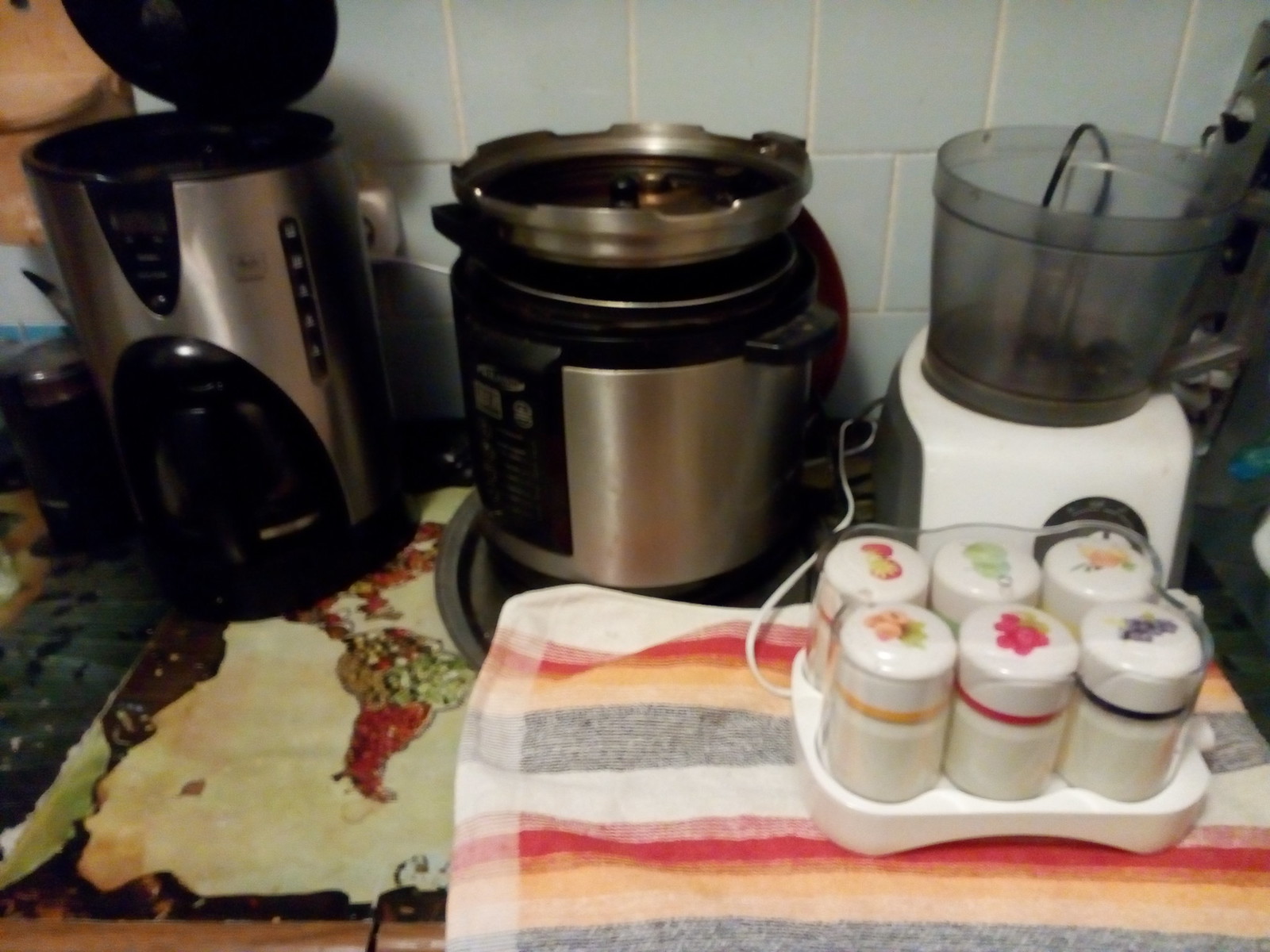This is a detailed color photograph of a kitchen countertop featuring several appliances and storage containers. On the left, there is a silver kettle with black accents. In the center, there is a silver metal jug, which might be a pressure cooker, with its lid open. To the right, there is a food processor with a dark gray, clear plastic cylindrical container on a white base. All these appliances are situated on a countertop against a backdrop of baby blue tiles with white grout.

In the bottom right corner of the image, there are six white cylindrical jars with fruit and floral patterns, including detailed drawings of grapes, strawberries, peaches, and other colorful designs. One jar features a peach-colored fruit, another green with blue accents, and another red with a beige or yellow central design. Additionally, to the right, there is a red, orange, and black striped tea towel.

Also visible on the countertop is a cutting board with a map of the United States and parts of South America, colored with splotches of red, green, maroon, and brown, with the USA highlighted in red and orange. The overall scene provides a vivid snapshot of a well-used and functional kitchen.